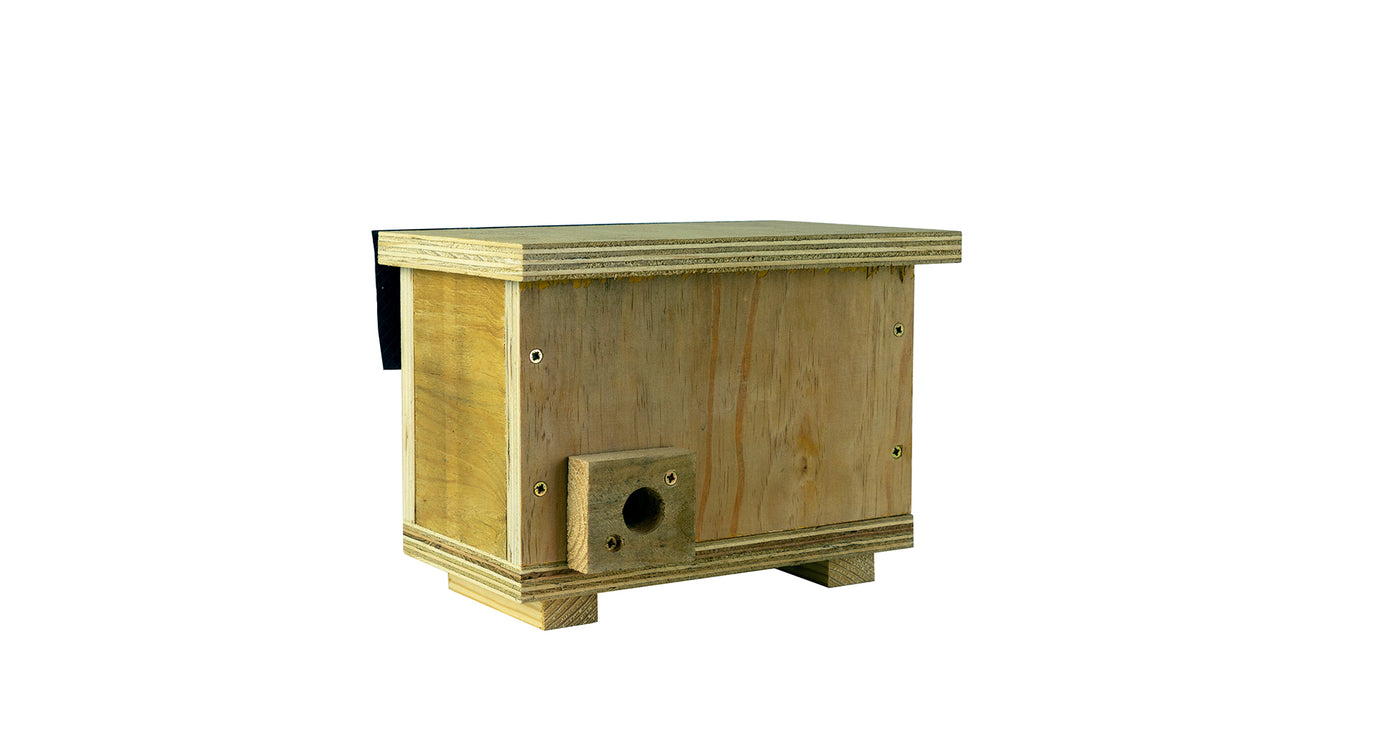The image displays a small, tan-colored wooden box, possibly constructed from plywood. Measuring approximately four inches tall and five inches long, the sides are secured with visible Phillips screws, and although the top is partially obscured, it's evident that it is also made of plywood, likely affixed in a similar manner. In the lower left-hand corner, there's a circular hole, suggesting a potential function as a birdhouse, albeit suited only for small birds. This hole is reinforced with an additional wooden block, held in place by a couple of screws. The box is elevated slightly above the surface it's placed on by wooden slats at each end, each about three-quarters of an inch thick. The image is set against a plain white background, highlighting its craftsmanship and the simplicity of the design.